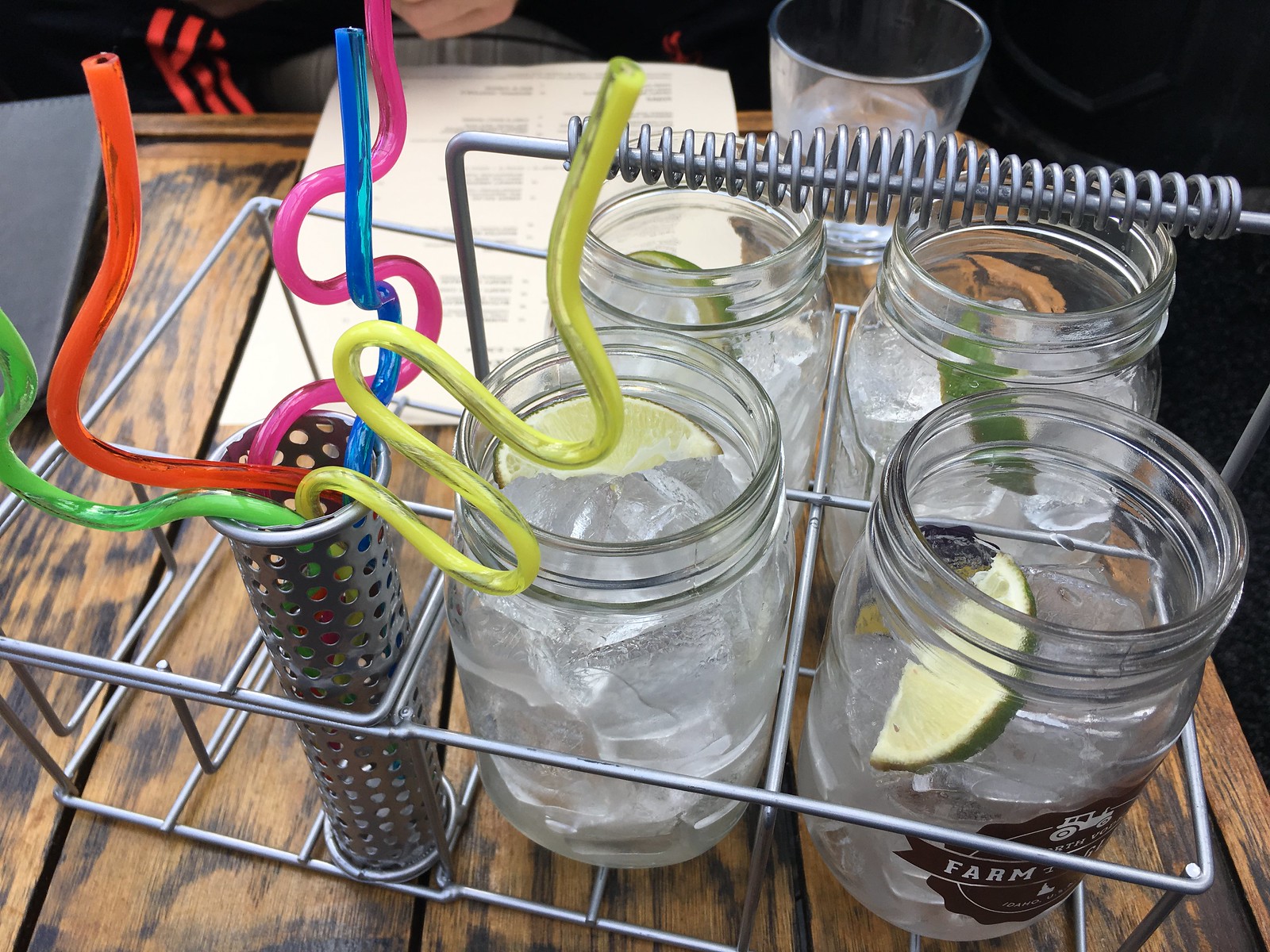This photograph captures a rustic scene with a detailed arrangement on a dark wooden table with prominent black grain patterns. Central to the image is a metal wire basket, segmented into four sections, each holding a clear glass mason jar filled with ice and topped with a slice of lime—green on the outside and yellow inside. These jars likely contain water or another clear liquid. Adjacent to this setup, there is a tall, silvery cylindrical container with perforations that house five colorful, bendy straws; they spiral in various directions and come in green, red, pink, blue, and yellow. 

In the backdrop, a white rectangular menu with black text suggests a restaurant setting. An empty round glass cup can also be seen behind the basket. Additionally, a white person's hand is visible near the cup and menu, wearing pants adorned with red stripes on a black background. Notably, the front mason jar features a sticker displaying a tractor and the word "farm" in white letters on a black background, subtly hinting at a rustic or agricultural theme.